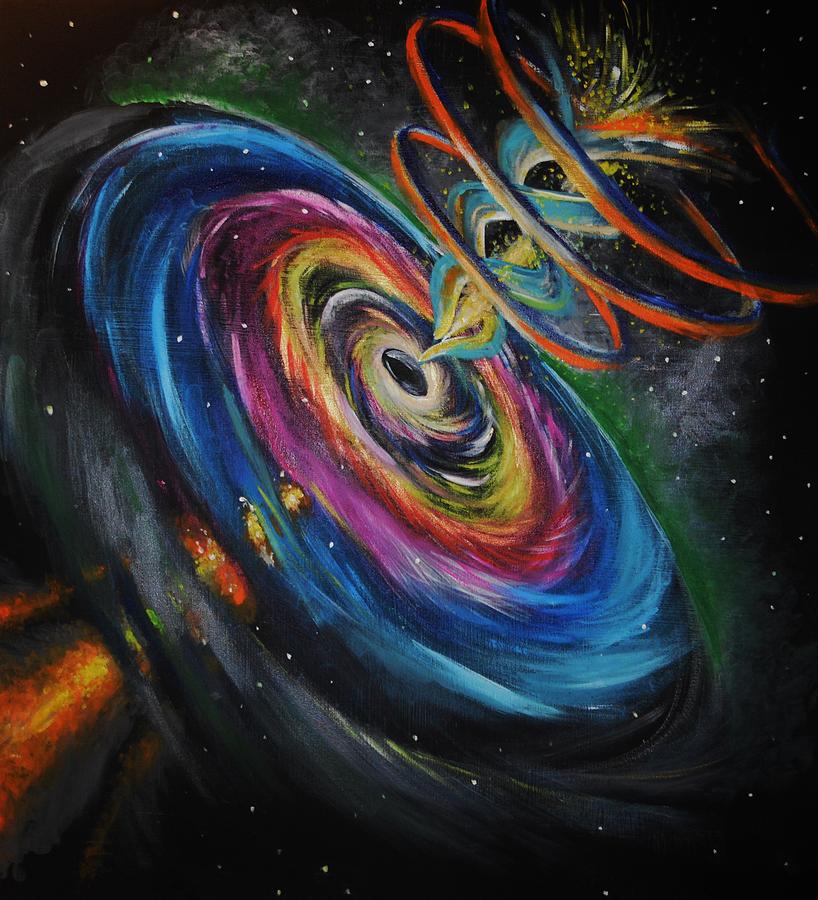The image is a very colorful and bright abstract piece of art, set against a black background resembling a starry outer space. Central to the composition is a vibrant, swirling vortex, reminiscent of a black hole or a cyclone, featuring layers of blue, purple, red, and yellow spiraling inward to a deep black center. Surrounding this colorful black hole are intricate swirls and patterns that evoke the motion of objects being sucked in. To the left, an orange and yellow trail, resembling a shooting star or fiery column, moves towards the black hole. Additionally, a DNA-like strand composed of light blue, green, yellow, and white, with three distinct turns, emerges from the top, framed by circles of red and dark blue. This dynamic and vivid artwork, possibly created with oil pastels, captures the intense and otherworldly energy of a cosmic event.